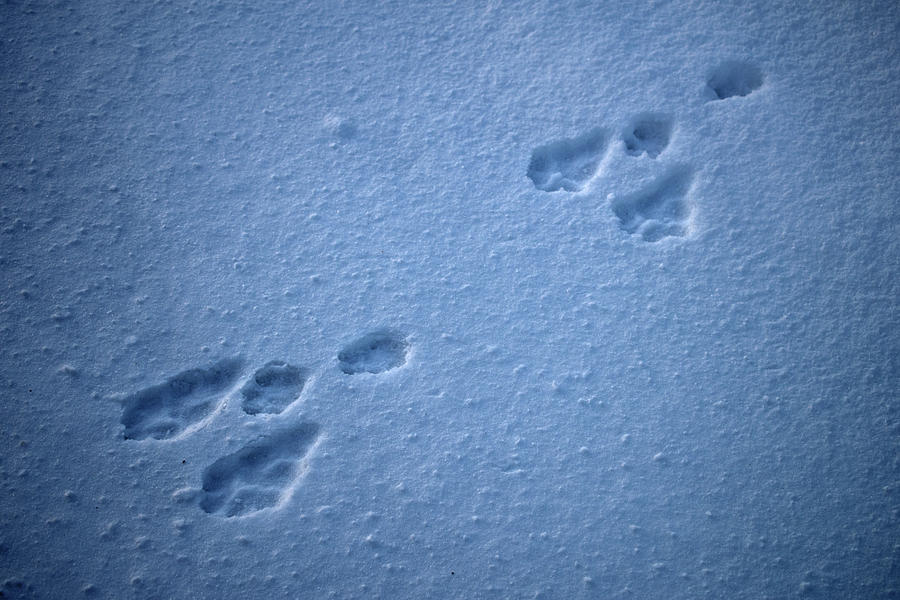In this close-up photograph taken from about a foot to a foot and a half above the ground, we see a pristine layer of snow with two meticulously aligned sets of animal footprints. The snow, while largely flat, has subtle, natural undulations and a bluish tint, indicative of dimming daylight in a cold climate. Each set of prints consists of four distinct depressions: two larger, ice cream cone-shaped impressions, and two smaller, roughly circular ones. Both sets of footprints are symmetrically spaced about five to six inches apart, suggesting the trail of an unidentified animal. The photograph's focus is solely on the footprints and the textured snow beneath, offering no other elements to distract from the serene, cold beauty of the scene.